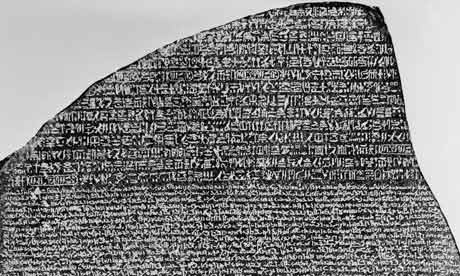The image is a black-and-white photograph of an ancient stone tablet with inscribed writing. The stone, which appears to be dark in color, has a rounded, arced top reminiscent of a shark's fin and seems to have been broken at some point. The inscriptions cover both larger pictographs in the upper three-fifths and smaller script beneath, all in a lighter color against the dark stone. The script, which is not in English, appears to be an ancient form of writing, possibly pictographic. The stone is visible along the lower and left borders and partially along the top and right, suggesting the image is cut off at the stone's base. The overall background of the image is light gray.